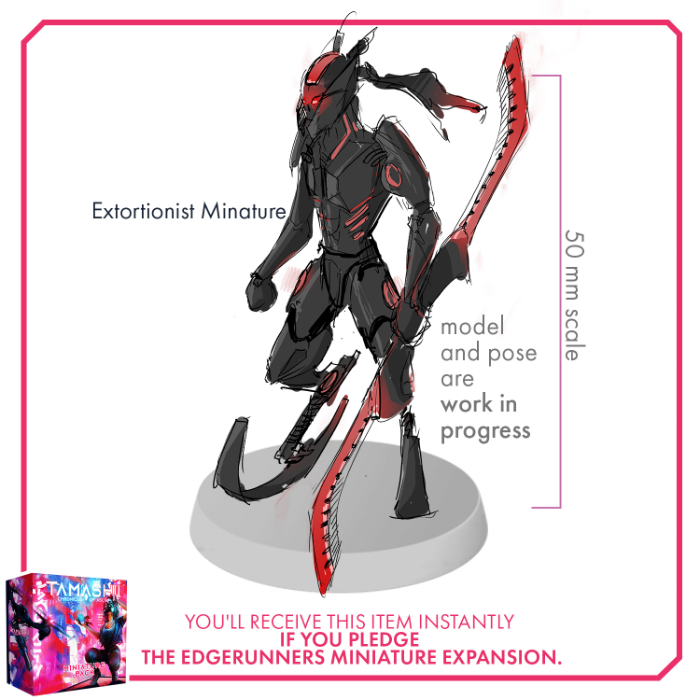The image depicts a hand-drawn sketch of a black robot adorned in futuristic, cybernetic bionic armor accented with red lines. The robot wears a mask with red markings and holds a very long red shawl, which is taller than the robot itself. Both legs are replaced with metal, curved legs, enhancing its mechanical appearance. The left side of the image features a label reading "Exhaustionist Miniature," while on the right side, it includes a note stating "model and pose are work in progress" along with a measurement scale indicating the height from the top of the robot to its neck is 50mm. The entire image is framed by a red square border, suggesting it might be a promotional photograph for a miniature toy, potentially from some form of media or product line.